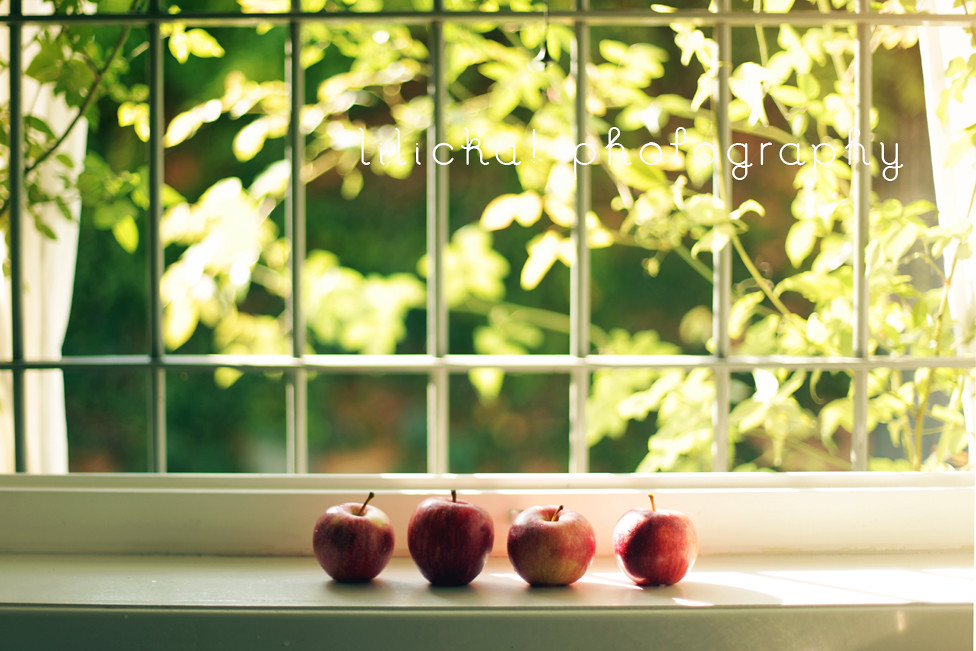This photograph captures a vibrant scene featuring four ripe red apples neatly arranged on a white, possibly wooden, windowsill, with their stems prominently displayed. The barred window through which sunlight pours in frames the background, casting a bright glow that enhances the green hues of the leaves and branches outside. The leaves, bathed in the sunlight, are a vivid yellowish-green. Despite the clarity of the scene, a watermark-like white text is overlaid in the upper right corner. The text appears loopy and faint, and while difficult to decipher, seems to end with "photography" or "of Graffy." The combination of the bright light and the white lettering over the foliage makes the inscription challenging to read. Overall, the contrast between the sunlit green outside and the tidy arrangement of apples on the white sill creates a crisp, lively image.